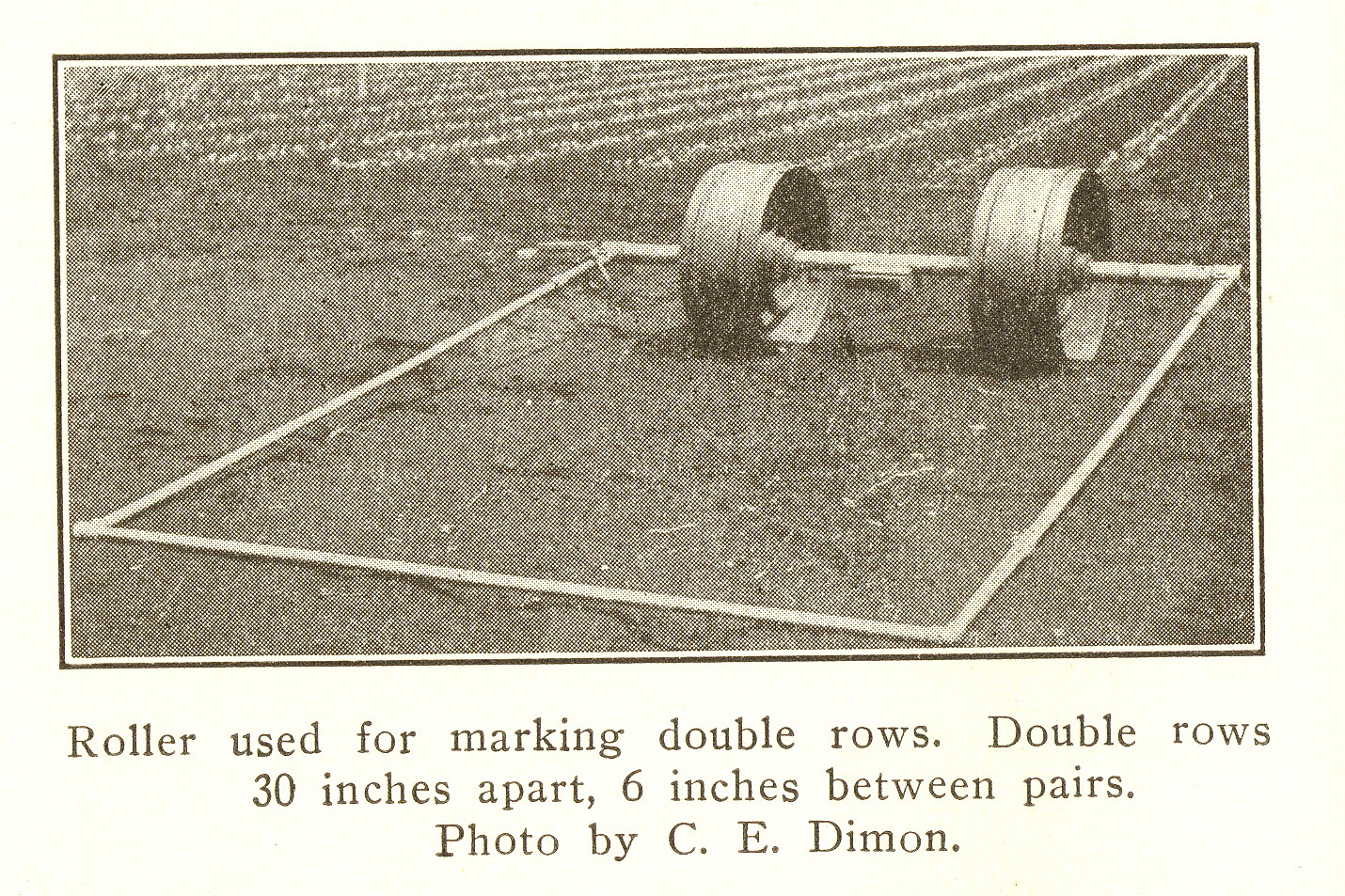This black and white photograph depicts an agricultural scene with a dirt field in the background featuring rows of newly planted crops. In the foreground, there's a box-like frame structure attached to two large metal wheels. This contraption resembles a barbell with weights but serves as a roller used for marking double rows in the field. The mechanism highlights rods and rollers arranged in a square formation. The text below the image reads: "Roller used for marking double rows. Double rows, 30 inches apart, 6 inches between pairs. Photo by C.E. Diamond."